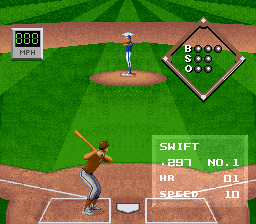The image is a screenshot from a retro-style video game, resembling a baseball game. The screen has a squarish shape, reflecting the simplicity and graininess of graphics typical of 20 to 30 years ago. From the perspective behind the batter, we see a baseball field with distinct dirt and green striped grass. The batter, positioned to the left of the white home plate, wears gray pants, a burgundy shirt, and a matching helmet while holding a bat. Directly opposite, the pitcher stands on the mound in white pants and a blue top. In the top left corner, a gray box displays "000" in green digital font above "MPH" in black. The upper right shows a diamond-shaped diagram tracking balls, strikes, and outs with the letters B, S, and O. Additionally, the bottom right corner has a translucent panel with details such as "SWIFT," ".297," "No. 1," "HR01," and "Speed 10." This image captures the essence of a vintage baseball video game in an engaging and nostalgic manner.